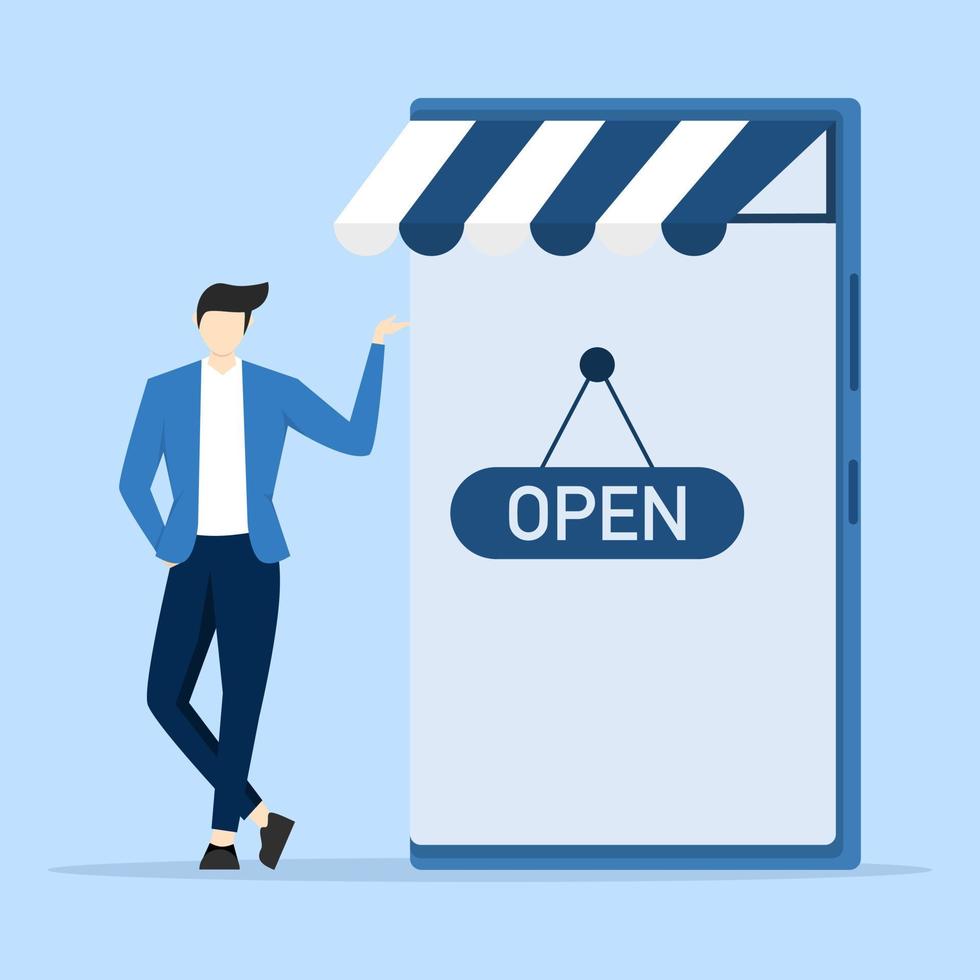The image is a vertical rectangular, digitally designed graphic with a light blue background, focusing on two main elements: a faceless cartoon figure and a storefront. On the left side, the faceless male figure, with a peach-colored face and hands, has black, swooped hair reminiscent of Elvis, and is dressed in a blue blazer over a white shirt, dark blue pants, and black shoes. He appears to be pointing toward the building on the right. The building's window is prominently placed from the middle to the right side of the image, featuring a blue outline on the top, bottom, and right edge. Above the window, a blue and white striped awning adds a sense of dimensionality. In the center of the window, an oval, dark blue "Open" sign with white lettering hangs from a blue peg, underscoring the welcoming nature of the storefront. The simple yet clear use of iconography conveys the scene with a professional, minimalist aesthetic.